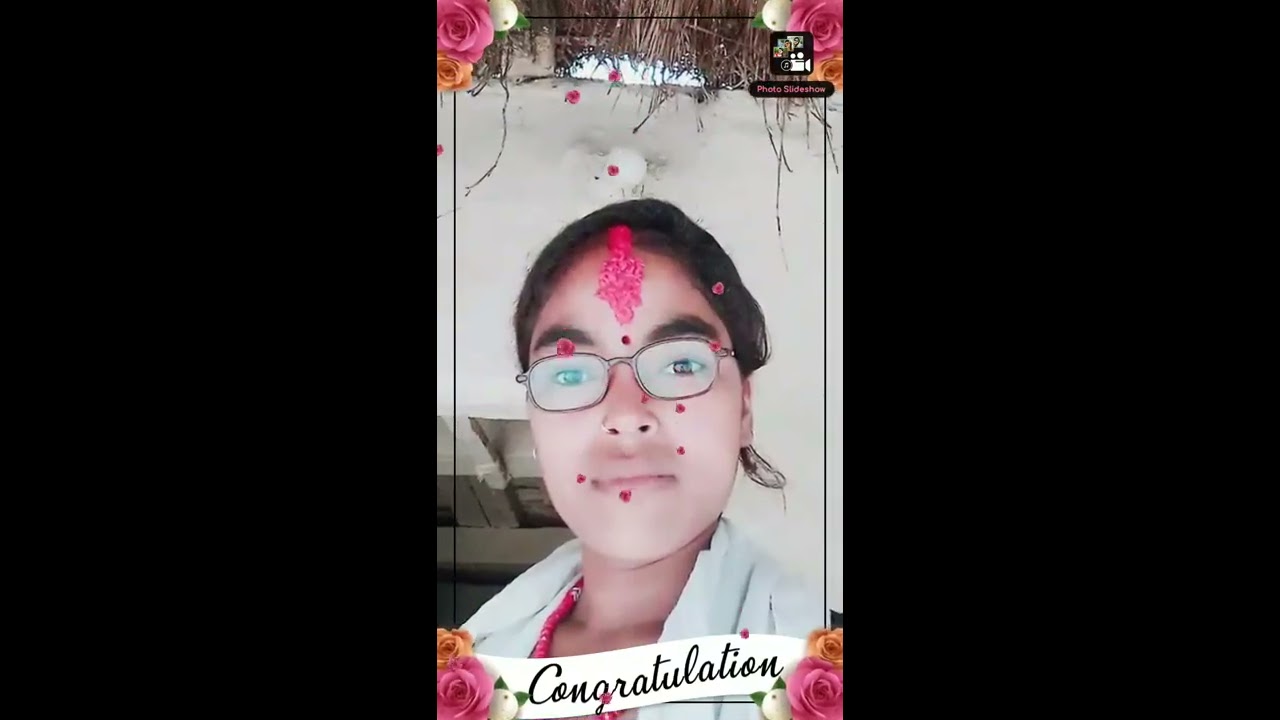The photograph is divided into three vertical sections, each two inches wide, with the outer panels in black and the central panel featuring the image. The central panel displays an edited photograph of a woman looking directly at the camera against a white wall. 

She has black, slightly pulled-back hair, oval black glasses, and a nose loop piercing on the left side. A pink beaded necklace adds a pop of color to her white shirt. The woman’s face and attire are adorned with animated pink and orange roses, some forming a pinstripe border around the photograph and others scattered as a filter effect over her skin and clothing. 

In the top right corner of the photograph, there’s a logo for an app, possibly named "Photo Slideshow," enhanced by additional flowers at the corners. Bottom of the photo displays a white banner with the word "Congratulations" in cursive, flanked by floral decorations. A white balloon with a red tip also appears to be floating behind her, adding to the festive ambiance.